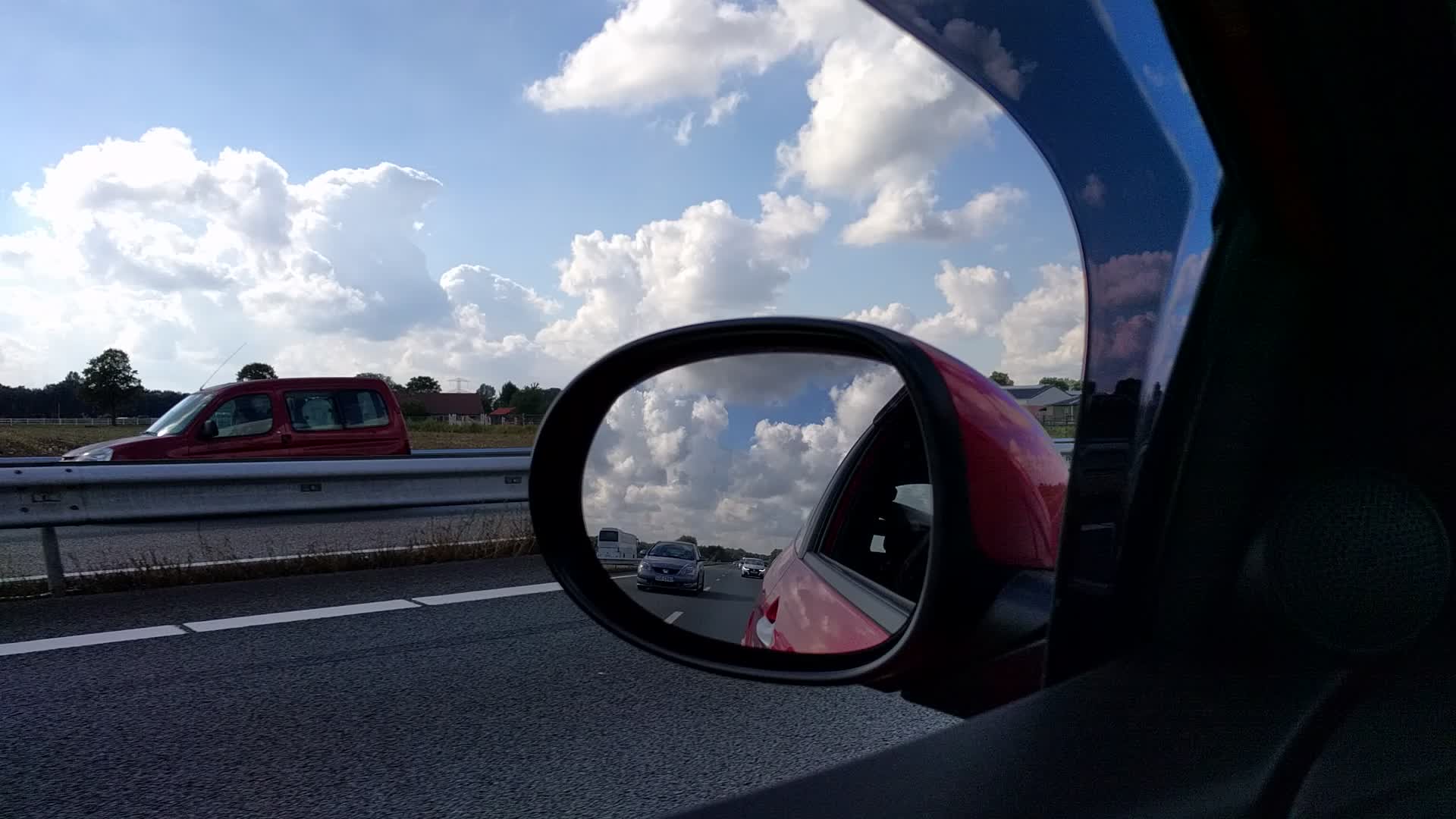The photograph is taken from the driver's side of a vehicle, capturing a detailed scene through the side mirror and outside the window. The car itself appears to be a darker red or maroon color. Reflections from a light source are visible on the mirror's surface, enhancing the image's depth. In the side mirror, a vehicle can be seen in the left lane, another car is trailing behind, and several vehicles are visible moving in the opposite direction.

Outside the mirror, the opposite lane of traffic is separated by a guide rail, which has a galvanized, bluish-gray tint. A dark red vehicle is also seen driving in the opposite direction, adding contrast to the scene. Central to the image, there is a patch of greenery on the ground, bordered by trees. The structures captured in the image include a building with a white exterior and a dark brown or reddish roof, positioned in the middle background. Additionally, on the upper right corner of the side mirror, part of another structure with a tan-colored roof is visible.

The sky is clear with light blue hues, scattered with white clouds, lending a serene backdrop to the highway scene. The fog lines on the road are clearly defined, marking each direction of traffic efficiently.